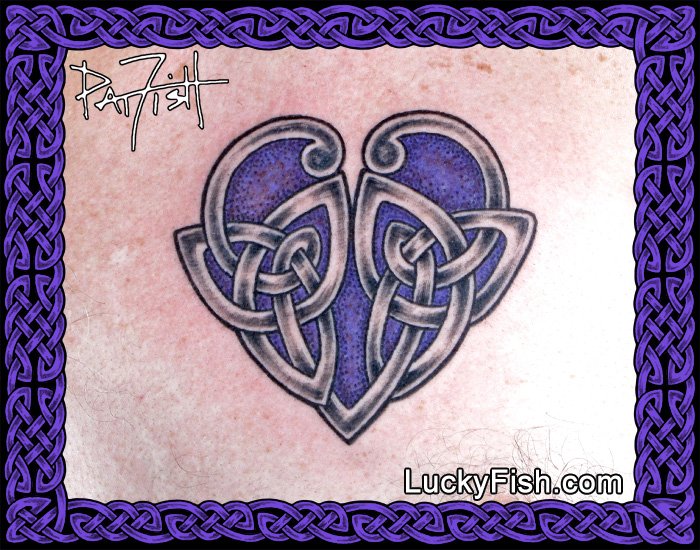This is a high-quality color illustration of a Celtic knot-style heart design. The heart, which features a detailed black and gray outline, is intricately woven and filled with blue and purple accents. Surrounding the heart is a dark purple Celtic knot border, which elegantly frames the central design. The background of the image is a light purplish-pink, trimmed and outlined in black, enhancing the overall aesthetic. In the top left corner, the text in white reads "Pat Fish," while in the bottom right corner, it states "luckyfish.com," both indicating the artist and website associated with the artwork.